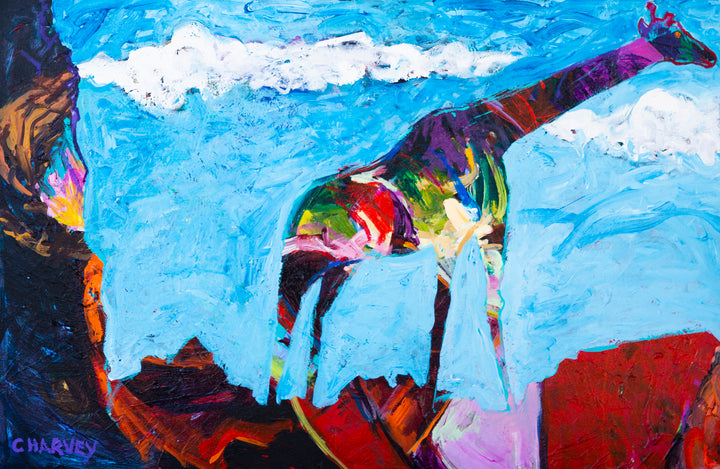This vibrant painting, signed by C. Harvey in blue in the lower left corner, features a multicolored giraffe standing against a bright blue sky adorned with fluffy white clouds. The setting appears to be a desert landscape, with large rocks in the distance painted in shades of orange, red, and black. The giraffe’s face is black with a striking red eye, and its long neck transitions from dark hues of black, purple, and blue at the top to brighter reds, yellows, greens, and purples lower down, finishing with touches of white. The ground beneath the giraffe is a painted red, with one front leg standing on a pink splotch. Behind the giraffe, there is a rock face characterized by a mix of black and blue colors, punctuated with vibrant yellow and orange highlights. The detailed brush strokes and vivid color palette make this piece a striking depiction of the majestic animal in an imaginative, surreal environment.